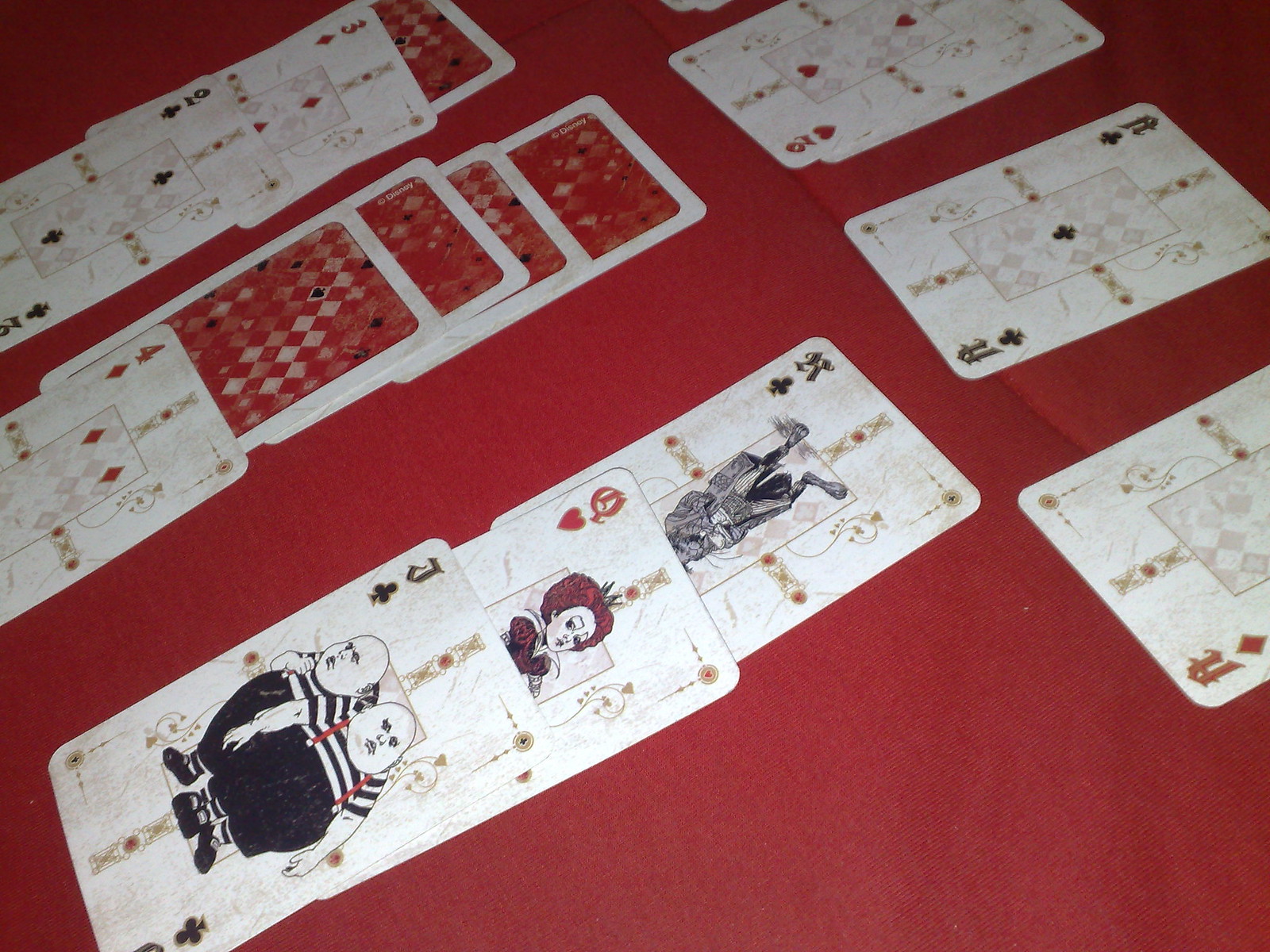A deck of unusually artistic playing cards is spread out on a cranberry-red tablecloth, suggesting a game of solitaire in progress. The cards feature highly stylized, almost surreal illustrations reminiscent of "Alice in Wonderland" characters, diverging significantly from traditional playing card designs. Notably, the face cards, including the King, Queen, and Jack, sport these unique illustrations, while some cards, like the Ace of Clubs, display only the symbolic club without additional figures. The back of each card showcases a checkerboard pattern in varying shades of red and white, interspersed with small symbols of hearts, diamonds, clubs, and spades, adding to their whimsical charm.